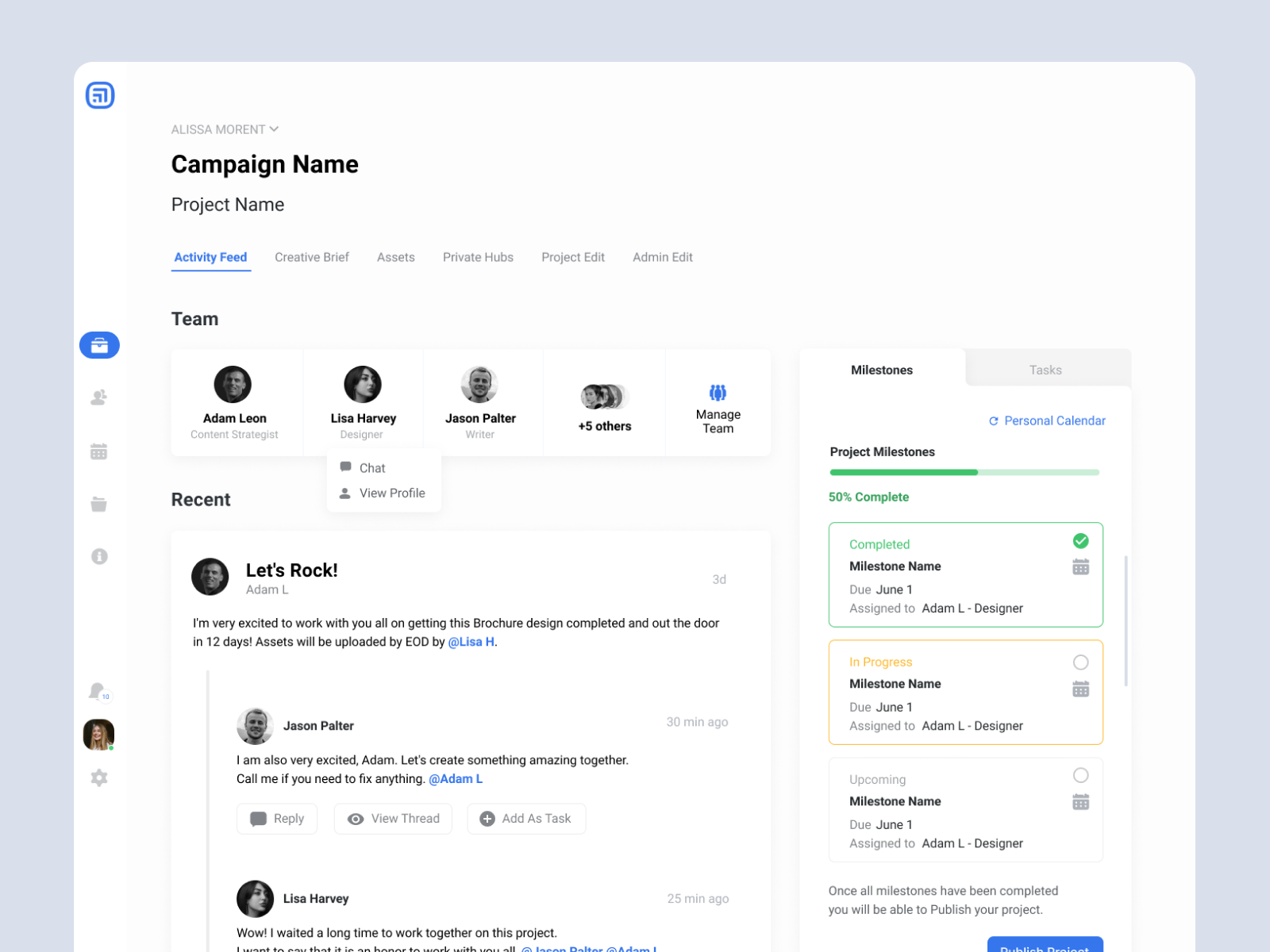**Image Description: Project Management Dashboard for Alyssa Morent's Campaign**

The image displays a project management dashboard enclosed in a gray box with various sections and details. At the top, heading text reads "Alyssa Morent," followed by labels for "Campaign Name" and "Project Name." Below these labels, there is a blue underlined link titled "Activity Feed."

Under the activity feed section, the following tabs are listed: "Creative Belief Assets," "Private Hubs," "Project Edits," and "Administrative Edit."

Beneath these tabs, there's a section titled "Team" that lists team members, including "Adam Leon" and "Lisa Harvey." Next to Lisa’s name, there are options for "Chat" and "View Profile." The list continues with "Jason Poulter" and mentions "five others." Adjacent to the team member names, there is an option to "Manage Team."

In the chat section, the conversation includes several messages:
- Adam L.: "Next, let's rock. I’m very excited to work with you all on getting this brochure design completed and out the door in 12 days."
- Lisa H.: "Assets will be uploaded by EOD."
- Jason Poulter: "I am also very excited, Adam. Let's create something amazing together. Call me if you need to fix anything."
- Lisa Harvey: "Whoa, I've waited a long time to work together on this project." (The message cuts off here.)

On the right side, the section titled "Milestones" includes project milestones:
- A progress bar indicates that the project is 50% complete, highlighted in green.
- A green checkmark marks a completed milestone labeled "Milestone Name," which was due on June 1st and assigned to Adam.
- An "In Progress" milestone, also due on June 1st and assigned to Adam, is highlighted in an orange box.
- An upcoming milestone, again due on June 1st and assigned to Adam, is noted.

The section concludes with a note stating, "Once all milestones have been completed, you will be able to publish the product."

This detailed and organized dashboard provides a comprehensive view of the project's status and team interactions, ensuring seamless collaboration and efficient progress tracking.